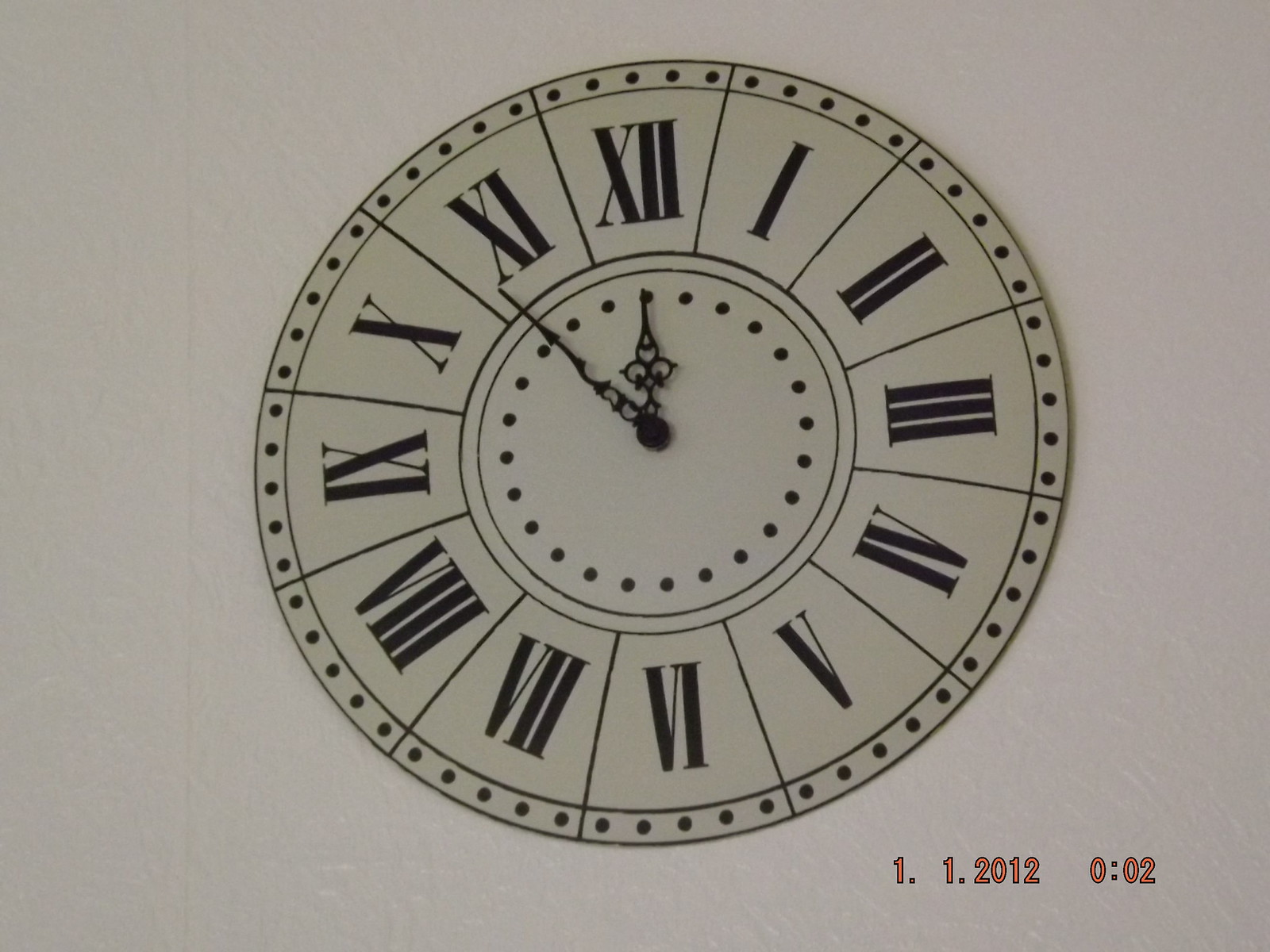The image features a round black and white wall clock displaying the time at approximately 11:54. The clock face includes Roman numerals for each hour, arrayed around the perimeter. Surrounding each numeral are individual dots organized into five-dot clusters along the edges of each numbered panel. Additionally, there is a circle of dots around the center, encircling the clock hands.

The minute and hour hands are black and pointed, clearly indicating the time. In the bottom right corner of the clock face, the date "1.1.2012" is displayed, accompanied by "0:02" just to its right. The clock is mounted on a white wall, which highlights the contrast with the off-white tone of the clock face. The overall image is slightly wider than it is tall, enhancing the horizontal aesthetic of the scene.